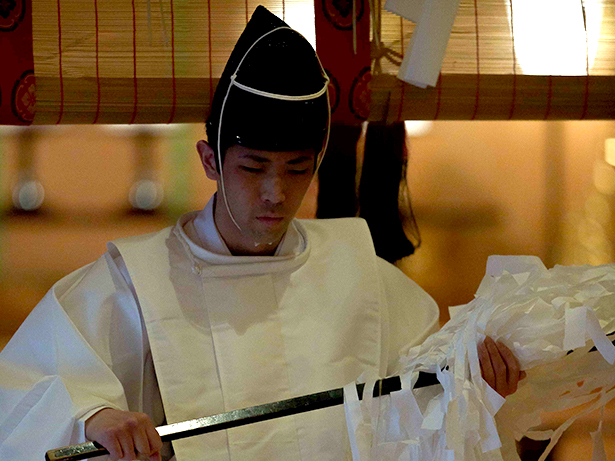The image captures a Japanese man in traditional attire, engaging with a black, shiny, rod-like object. He is shown from the waist up, wearing a thick, puffy white robe with expansive sleeves that add to his traditional look. He accessorizes with a pointed black hat, secured under his chin with a white string. The man appears concentrated on the task at hand, which involves working with what seems to be fringed white paper, possibly shredding or manipulating the material that is draped around the rod. The background features a slightly blurred brown wall, with hints of bamboo, adding an authentic cultural context to the scene. The image is brightly lit, capturing all details with clarity.